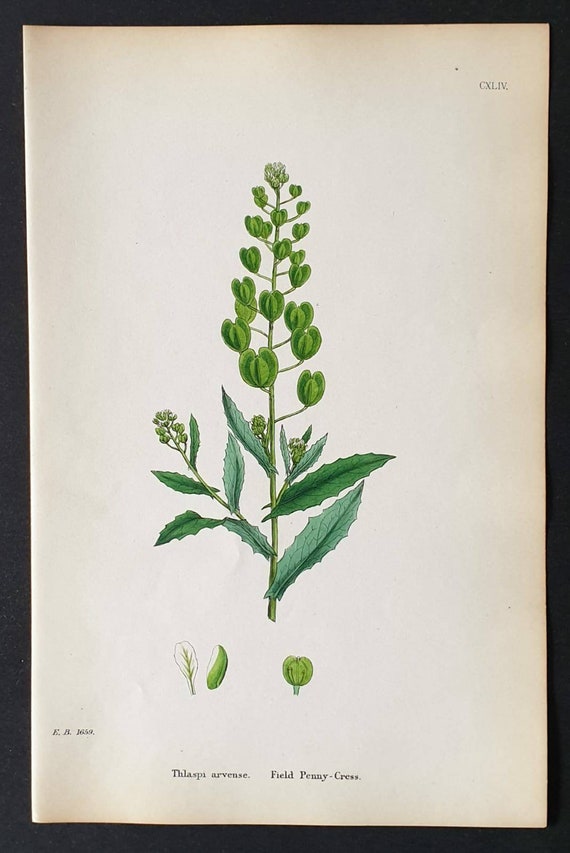In the photograph, a slightly discolored, old-looking rectangular piece of white paper is placed on a black surface. The focal point of the paper is a detailed botanical illustration of a green plant. The plant has a conical structure with a green stem and varying leaf shapes. Dark green leaves with ridged, pointy edges grow off the bottom of the stem, while lighter green leaves with a different shape are positioned higher up. At the top, small bulbs adorn the plant, reminiscent of a Christmas tree shape. 

Beneath the main plant illustration, three smaller individual drawings of different portions of the plant are displayed. At the bottom center of the paper, the scientific name "Thlaspi arvense" along with its common name "Field Penny Cress" are written. Additionally, small text on the bottom left reads "E.B. 1659." In the top right corner of the paper, the letters "CXLIV" are inscribed. The setting is bright, with natural lighting enhancing the clarity of the image.